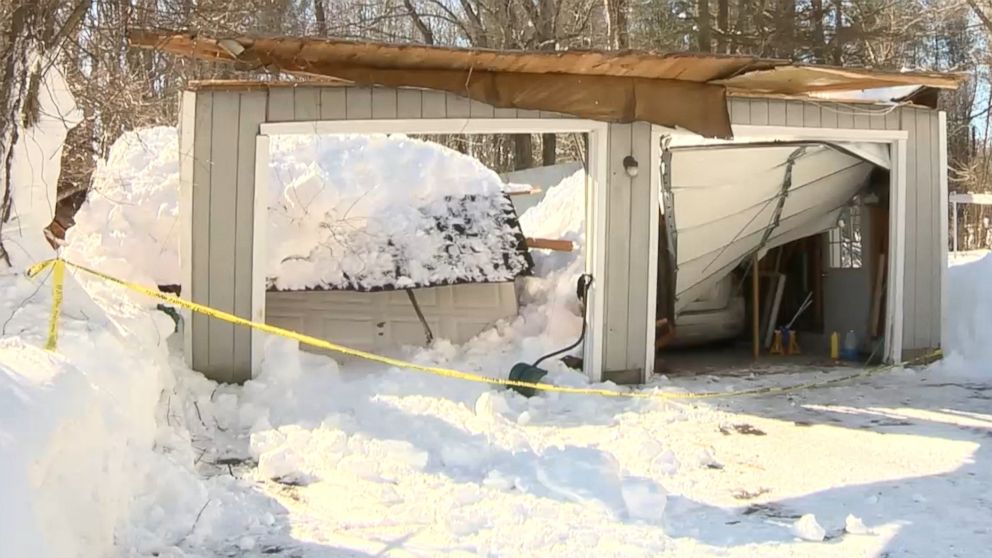The photograph captures a deeply damaged, tan-colored two-car garage in a rural, wintry landscape. The scene is filled with snow, indicating it is wintertime, and the surrounding area is populated with trees. The garage's roof has completely collapsed, with its brown remnants scattered among the debris. The structure's condition points to a severe incident, possibly an avalanche. Both garage doors are severely damaged; the left door is pushed in and mangled, while the right door hangs halfway down, twisted. Inside the garage, whose detailed contents are obscured, a car might still be parked in the right bay. A caution tape is strung across the garage entrance, indicating danger. A snow shovel rests against the garage side, near the pavement where the snow has been cleared, creating a stark contrast to the high snow piles around. Additionally, there's a light fixture situated between the two garage doors, hinting at the structure's functional past. The sunlight casts clear shadows across the scene, emphasizing the day's brightness amidst the devastation.